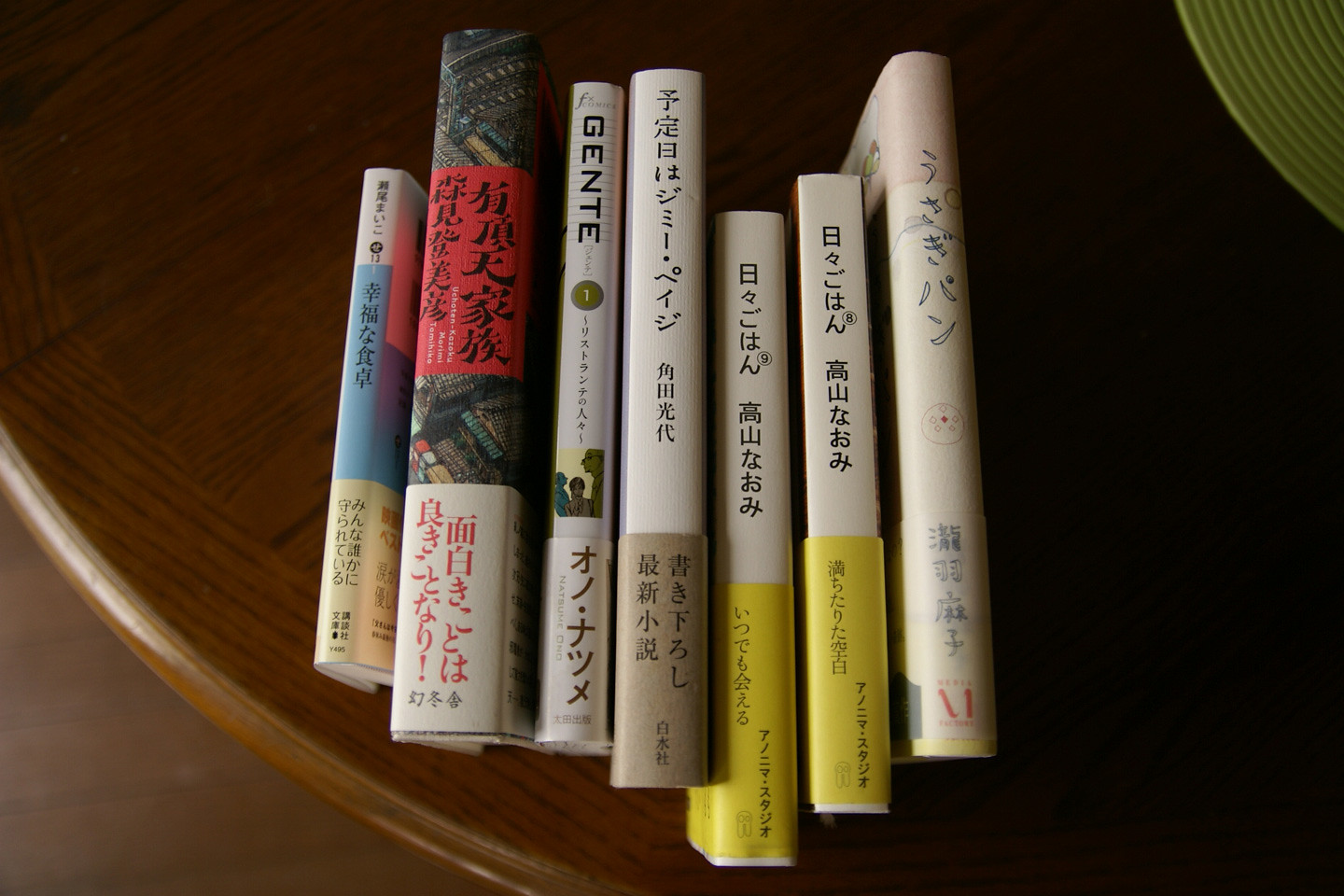The color photograph captures an indoor setting and focuses on a round, dark wooden table with an evident grain pattern, showcasing seven hardcover books stacked horizontally. The spines of the books, adorned with Asian lettering, face upward, creating a jagged edge both at the top and the bottom. Among the primarily Japanese titles, one book notably features the English word "GENTE" at the top of its spine. Two books have distinctive yellow labels covering the bottom third of their spines. A light dark brown floor is visible at the bottom left of the image, while a green table dish resides on the right. In the background, there's a hint of what appears to be a cityscape, or perhaps a Japanese town, adding depth to the scene.